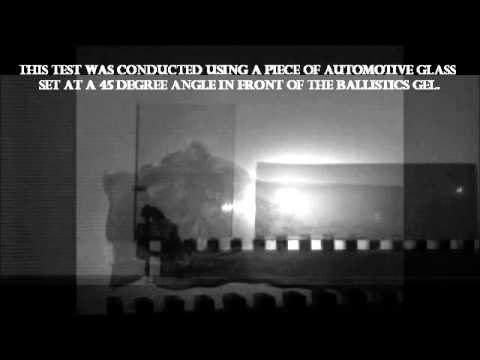The grayscale image features a blurry, indistinct view dominated by thick black borders at the top and bottom. The central area reveals a test setup involving automotive glass set at a 45-degree angle in front of ballistic gel, illuminated by a central light. The white, bold text at the top reads: "This test was conducted using a piece of automotive glass set at a 45-degree angle in front of the ballistics gel," spread over two rows. Despite the darkness, a faint pattern is discernible at the bottom, and there are also bridges extending from the off-centered left towards the right side, suggesting structural elements or reflections. The overall color scale of the image is a mix of black, white, and various shades of grey, contributing to the murky and indistinct atmosphere of the scene.